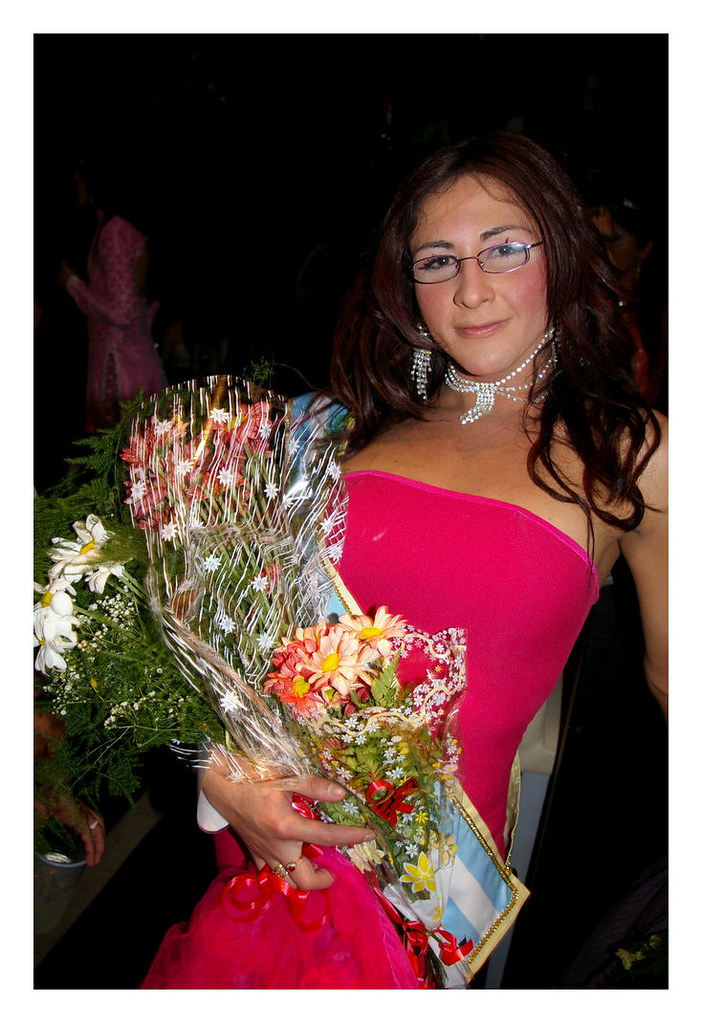This image captures a radiant young woman, likely around 19, with long, wavy, dark brown hair that extends slightly past her shoulders. She is smiling softly at the camera through her small glasses, her teeth not showing. Her outfit is a striking pink or fuchsia dress, resembling a crop-top or tube top without visible straps. Adorning her neck is a layered pearl necklace that drapes elegantly down, complemented by long, dangling pearl earrings. In her right arm, held close to her body, is a vibrant and diverse bouquet of multicolored flowers. The background is very dark and indistinct, making it challenging to determine if the setting is indoors or outdoors. However, there is a faint suggestion of another person on the left side, possibly a woman in a pink dress, though her features are hard to distinguish. The photograph conveys a focus on the main subject, who exudes happiness and elegance amidst the obscured surroundings.